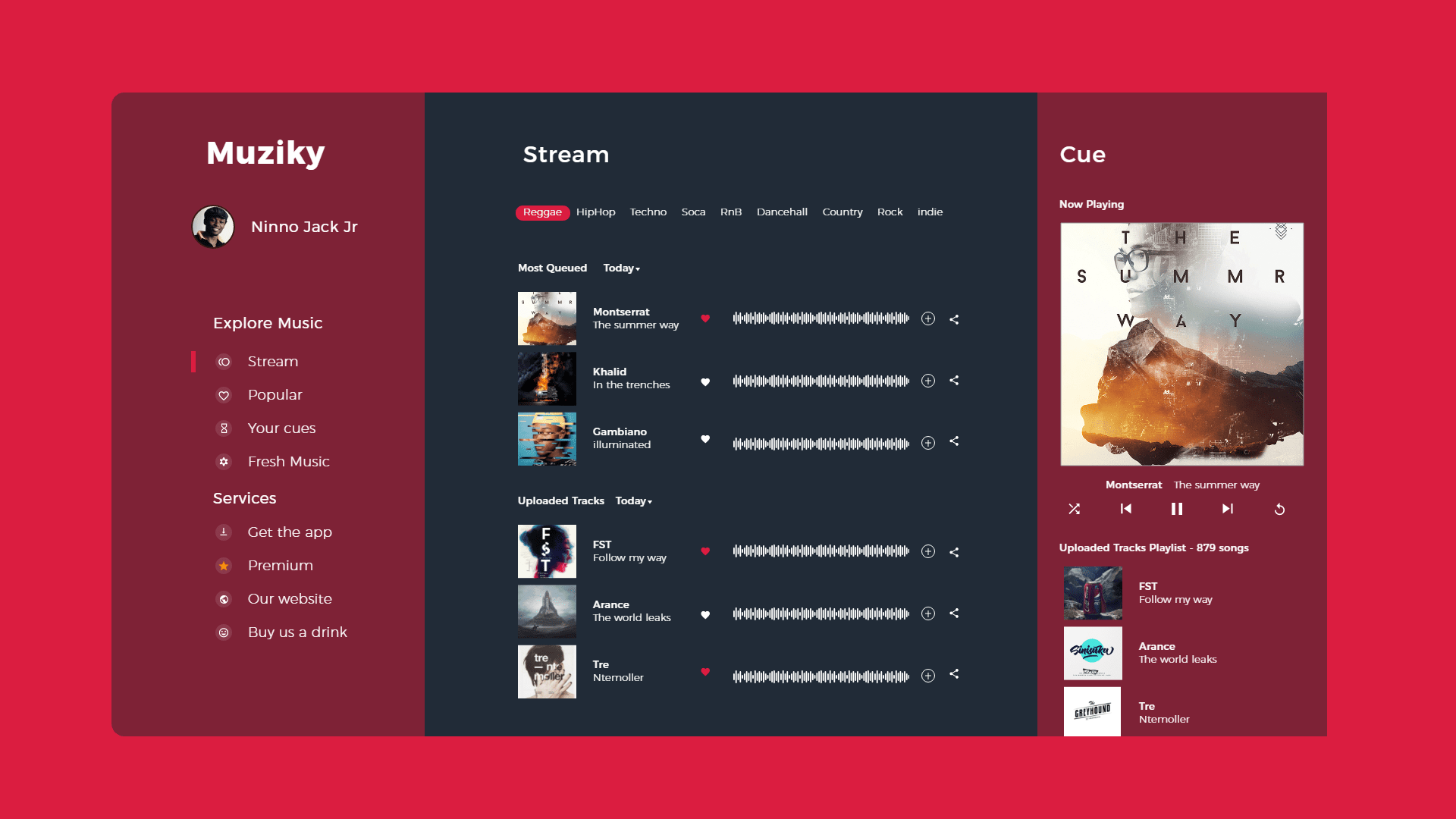The image is a screenshot of a computer screen interface, featuring a design with a bright red background. In the foreground, there is a large rectangular element bordered in red, divided into three distinct sections. 

The left section is a maroon red color, displaying text in white. At the top, the word "Musiki" is prominently featured. Below this is a circular image of a person along with their name. Underneath, there is a series of options listed under the heading "Explore Music," including choices such as Stream, Popular, and several others, totaling around five to eight options.

The middle section, which is black, is focused on streaming. It has several tabs at the top; the first tab is highlighted in red. This section contains six vertical rows, each with a small square image on the left, presumably album covers, and accompanying white text to the right of each image.

The right section, also in a maroon red color, is titled "QM Top." It features a square image that appears to be an album cover, predominantly white with a brownish-red design. Below the image, additional information is presented, though the specific details are not entirely clear in the screenshot.

Overall, the interface design is clean and visually segmented, allowing for intuitive navigation through musical content.